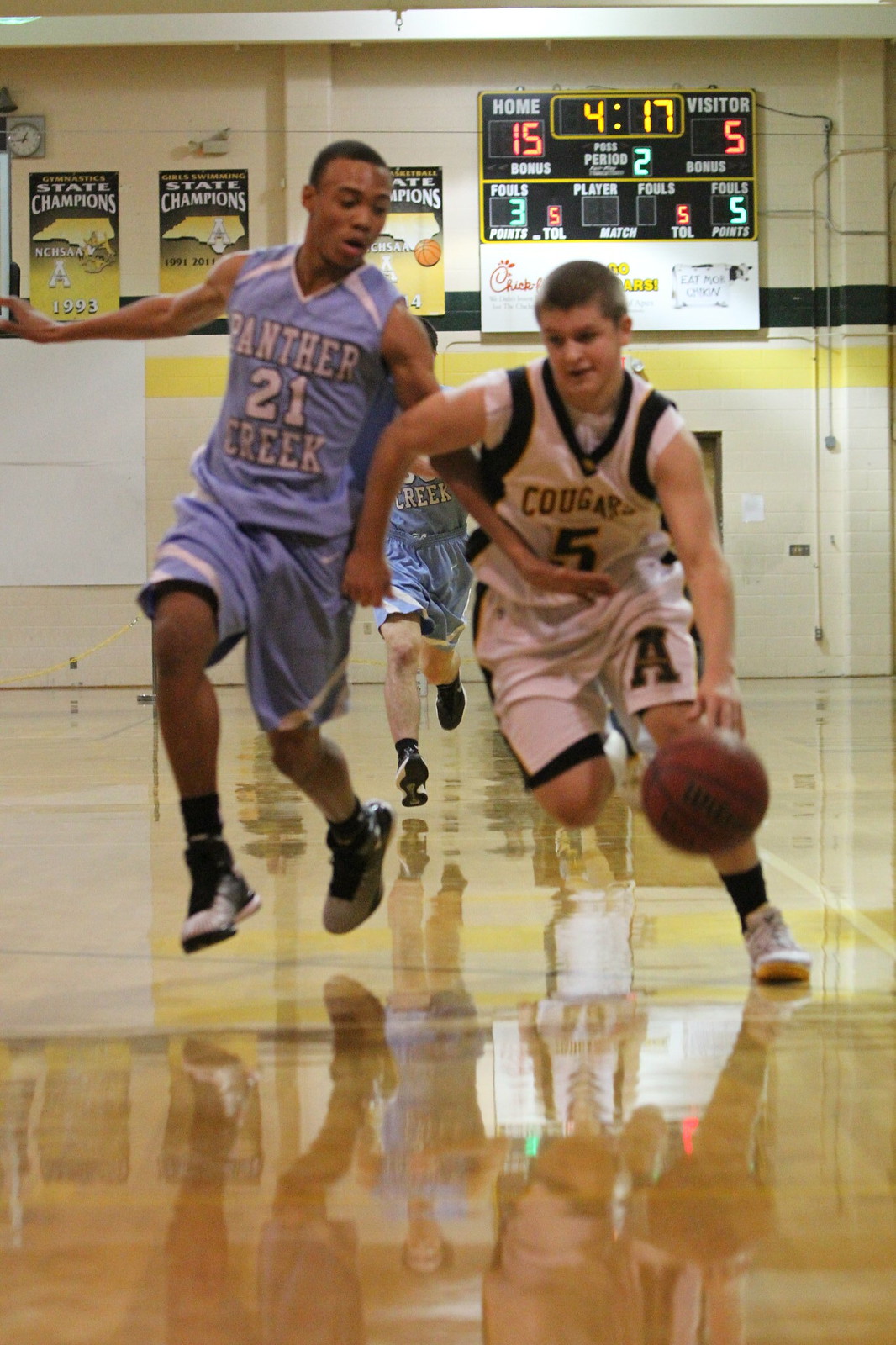This photograph captures a high school basketball game in the second period with 4:17 on the clock. The home team leads with a score of 15, while the visitor team, Panther Creek, trails with 5 points. The game is being played in a gymnasium, which has banners indicating state champion titles and a scoreboard sponsored by Chick-fil-A and others. Two players are prominent in the image: One from the Cougars, in white and black uniform, is dribbling the ball with a confident smile on his face. He is pursued by an African-American player from Panther Creek, wearing a light blue uniform with the number 21, attempting to block him. The home team has accumulated three fouls, while the visitors have five.